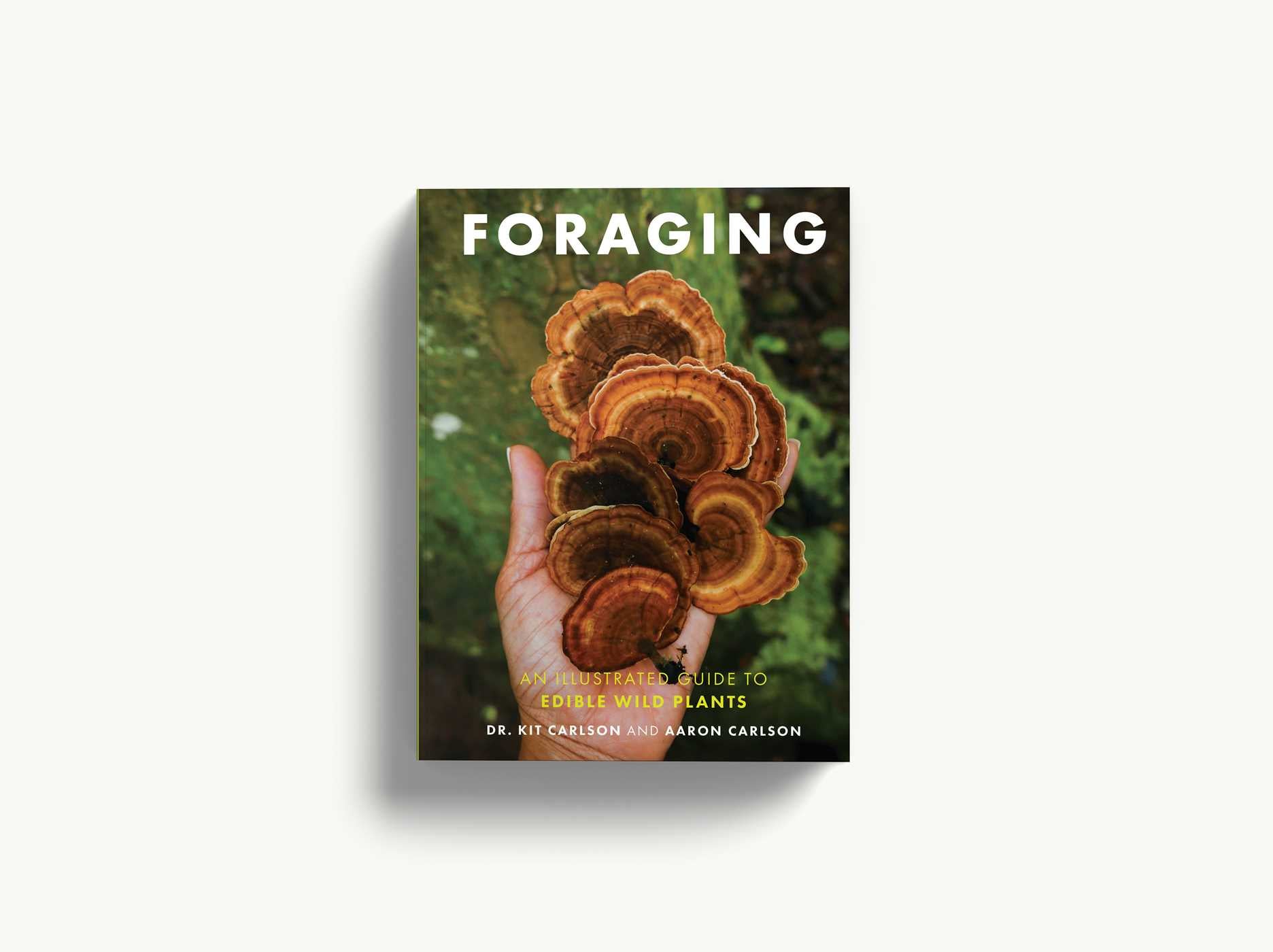The book cover features the title "Foraging" prominently displayed in white text at the top. Below, in yellow letters, it reads, "An Illustrated Guide to Edible Wild Plants." Further down, the authors' names, Dr. Kit Carson and Aaron Carson, are listed in white text. The central image on the cover showcases a left hand holding several brown mushrooms, differing in size, but all sharing a distinctive appearance reminiscent of the inside of a tree trunk, characterized by dark wood brown tones with some orange and red rings. The mushrooms are whole, not sliced, with visible stems. The background of the image is blurred, featuring green moss and possibly algae-covered rock, enhancing the natural foraging theme of the book. The overall setting of the book cover is laid against a minimalistic white background.